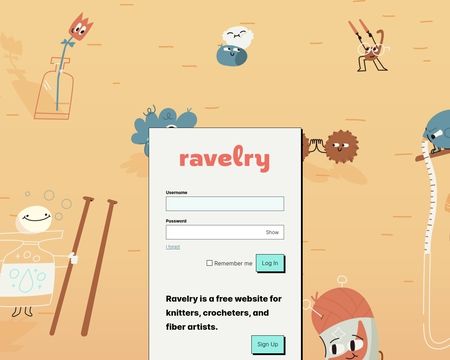A vibrant screenshot of the Ravelry website login page showcases an inviting and whimsical design. The background is a warm orange hue embellished with simple, artistic illustrations. Among these charming drawings, a vase with a rose, two smiling birds, a quirky crab wearing glasses, and a bottle seemingly clutching knitting needles stand out. Other partial illustrations add to the playful atmosphere, though their full details remain hidden.

At the center of the page, the Ravelry logo is presented in a stylish orange script. Below the logo, users are prompted to enter their username and password, with an option to remember the login information for future visits. The main action buttons, in a pleasant teal-green, offer choices to either "Log in" or "Sign up." A friendly note beneath the login fields describes Ravelry as a free website dedicated to knitters, crocheters, and fiber artists, inviting new users to join the community with a simple click.